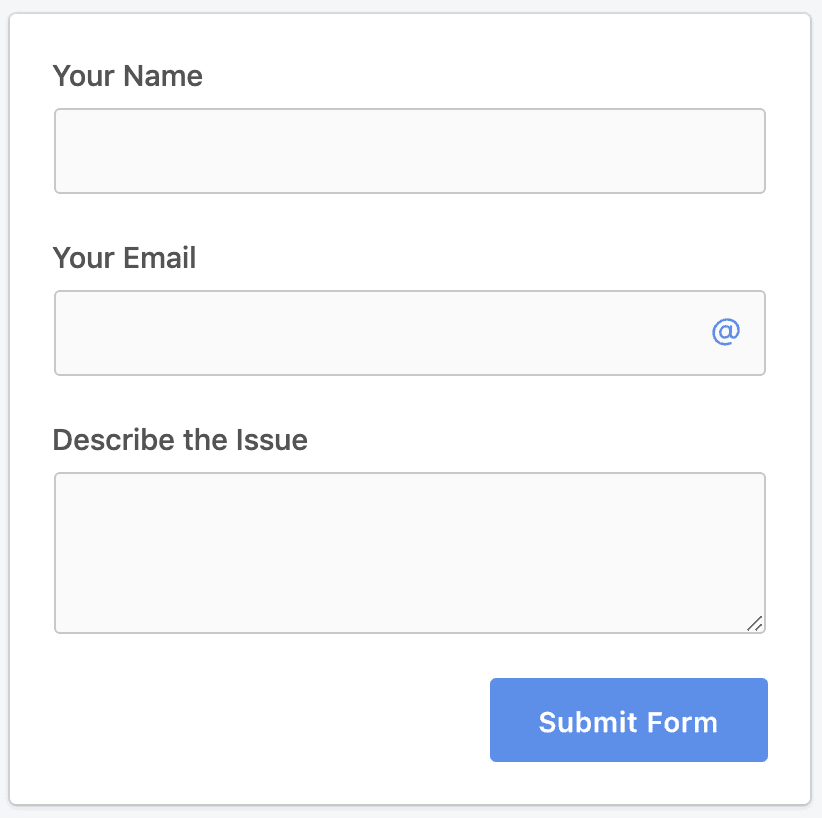The image is a minimalist design with a predominantly white background and a very light grey perimeter resembling a border. At the top left, there is a bold black text that reads "Your Name," with both 'Y' and 'N' capitalized. Below this is an empty horizontal rectangular input box, which features the same light grey color as the border behind its white interior. Further down, the text "Your Email" is written in black with capitalized 'Y' and 'E,' and no hyphen. There is an input bar below this, distinguished by a blue hyperlink '@' symbol, but it is otherwise empty.

Continuing downwards, the text "Describe the Issue" appears in black bold letters, with the 'D' in 'Describe' and the 'I' in 'Issue' both capitalized. Beneath this heading, there is a larger dialog box, which includes a stretch icon at the bottom right corner, but it remains unfilled. At the very bottom right of the image, there is a large blue "Submit Form" button with white text, with the 'S' in 'Submit' and the 'F' in 'Form' capitalized.